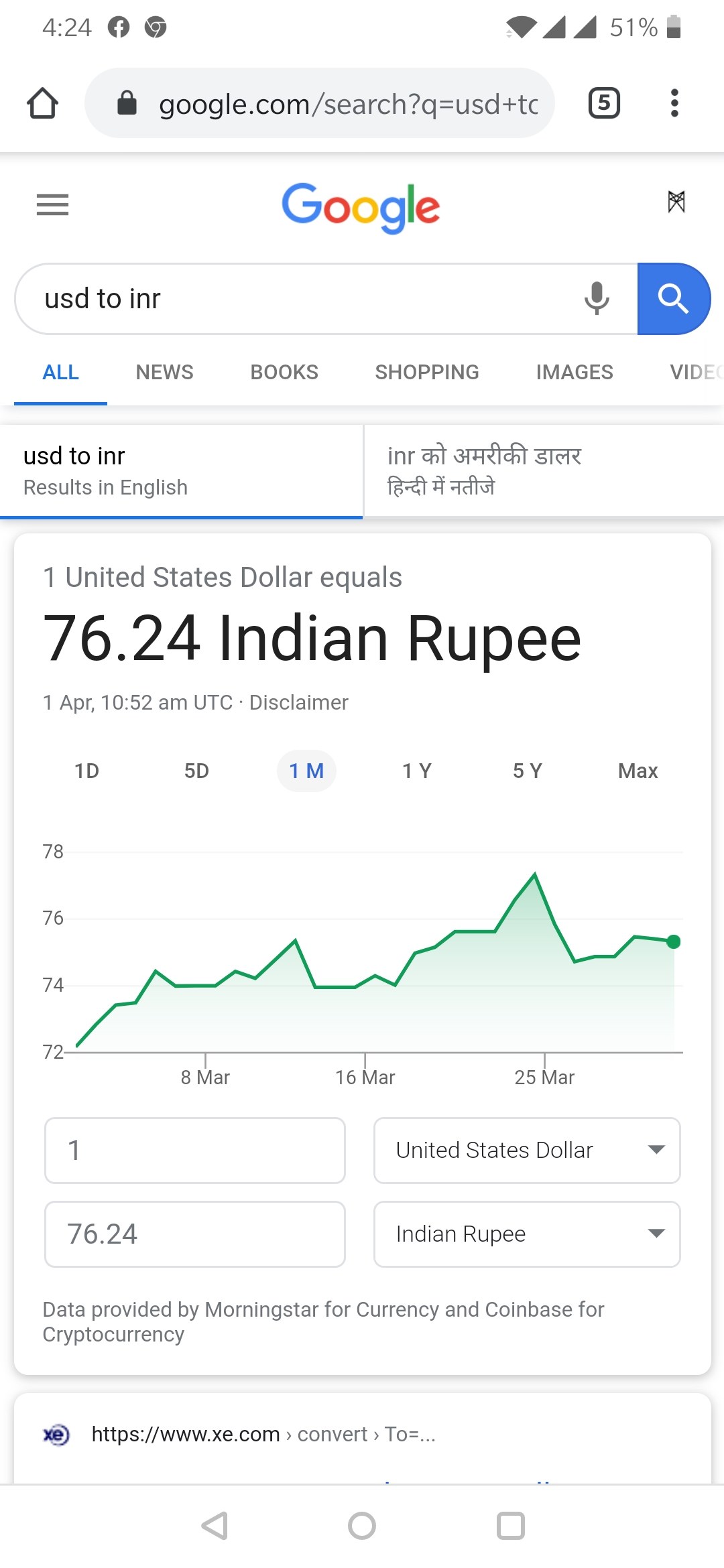This image depicts a smartphone screen displaying a Google search results page with a predominant white background. At the top, the status bar shows the time as 4:24 and the battery is at 51%. Below it is the gray search box with the Google homepage visible, displaying the iconic multicolored Google logo with a small black square containing a black number 5, and the three-dot menu icon beside a grey line. To the top right, there's an insignia resembling an 'M' intersected by an 'X'.

The search query seems to be related to currency conversion, specifically "USD to INR", and the results section is highlighted. Tabs for "All", "News", "Books", "Shopping", "Images," and "Videos" are shown with "All" being underlined.

The main result displays the exchange rate: "1 USD equals 76.24 INR," with a timestamp of "1st of April, 10:52 AM, UTC" indicated next to a disclaimer. The graphical data indicates currency fluctuations over selected time frames – "1 day", "5 days", "1 month" highlighted in blue, "1 year", "5 years", and "max". The dates "8th", "16th", and "25th of March" are noted below a trend line that peaks and then dips back down.

Further down, there's a section of smaller white boxes with gray print, the first containing "1 USD equals 76.24 INR" and data sourced from Morningstar for currency and Coinbase for cryptocurrency. A blue button marked with an 'X' and the URL "http://www.xz.com" is visible, leading to a service named "Conver". At the bottom are three small icons within a white box, potentially indicating additional navigation or functionality.